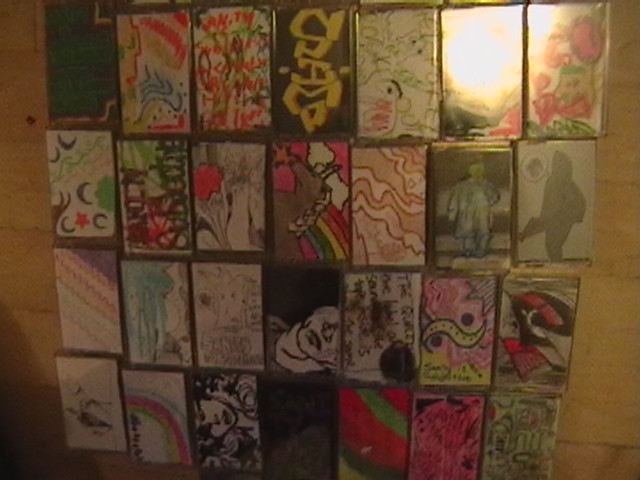This indoor photograph captures a vibrant, eclectic collage of what appears to be 28 cassette tape cases, each housing a unique piece of hand-drawn art. These miniature artworks are meticulously arranged in a grid pattern, four rows down and seven across, though one slot in the top left corner is conspicuously vacant. The diverse styles range from detailed and colorful illustrations to simple black-and-white sketches. 

For instance, among the varied pieces, there's a detailed depiction of a face on the bottom row, a silhouette of a person with a speech bubble on the second row from the top, and a dynamic composition of squiggly pink lines on the second row from the bottom. Other pieces include images resembling robots, shadows, and even potential drawings of celebrities or unicorns. Some artworks seem to incorporate writing, though the handwriting in thick marker is difficult to decipher due to the photo's low resolution and occasional glare.

The overall display exudes a vibrant array of colors and artistic expressions, set against what appears to be a wooden background. This intricate assemblage could very well be a collective project, possibly an assignment where each artist decorated a cassette tape case to reflect a personal or significant theme. Regardless, the collection distinctly showcases the unique creativity and individuality of its contributors, making it a visually captivating and thought-provoking montage.